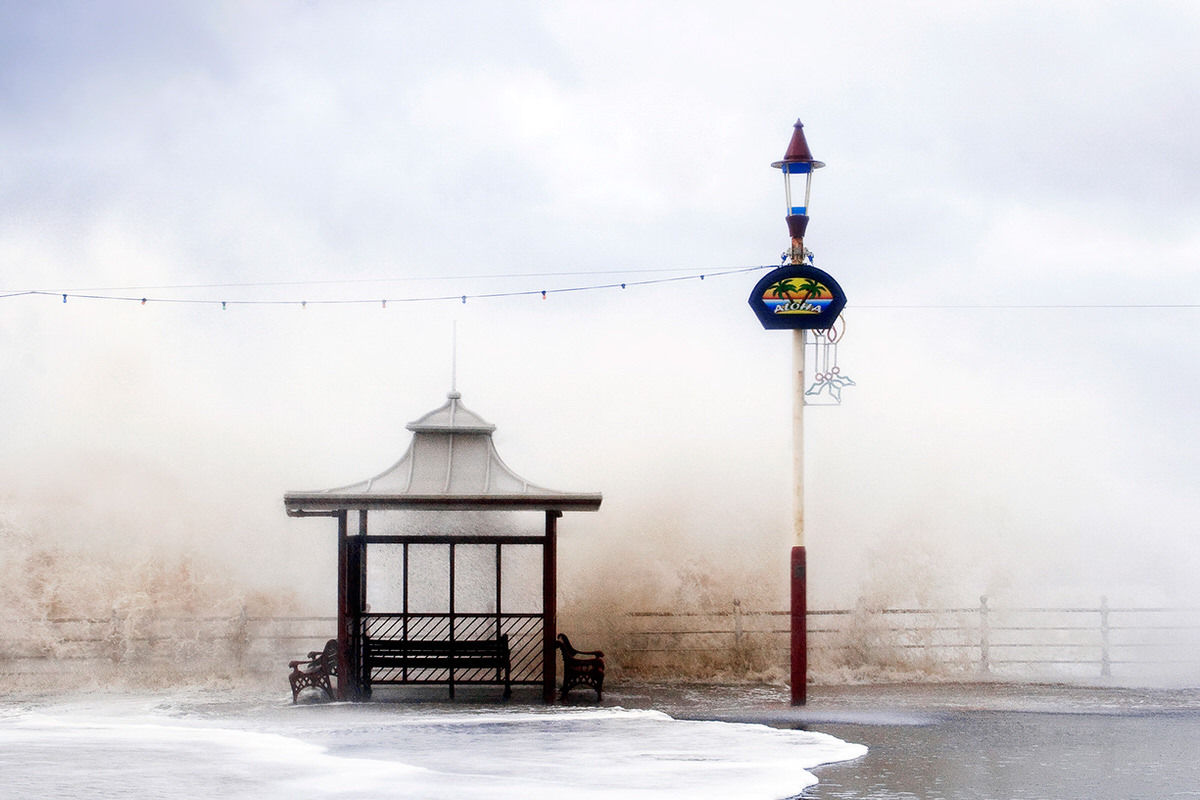This painting depicts a serene winter scene centered around a quaint gazebo. The gazebo is surrounded by three park benches—two positioned on the outside and one at the back. The ground in front of the gazebo is covered in patches of melted snow. In the backdrop, a fence extends across the width of the painting, partially obscured by a thick fog, contributing to the scene's serene, almost mystical atmosphere. A festive pole adorned with Christmas lights is visible, featuring an illuminated decoration of two candles. Adding a touch of tropical warmth to the chilly setting, two palm trees stand prominently, accompanied by the word "Aloha," suggesting a connection to Hawaii. Twinkling string lights are strung up around the gazebo, casting a warm glow despite the fog or snow that envelopes the scene.